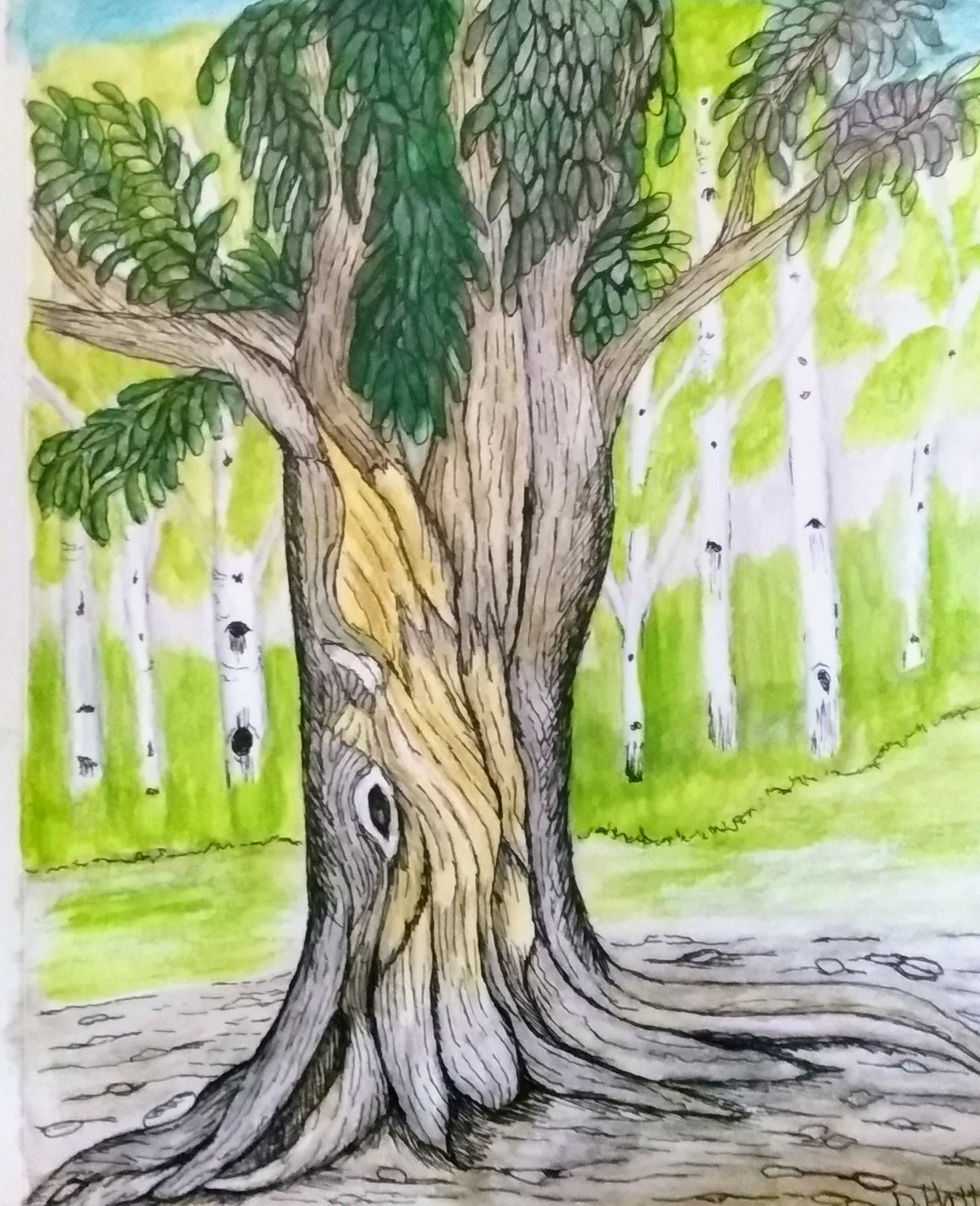The image depicts a detailed artist's rendering of an aged tree at the forefront, characterized by a slightly yellowed center trunk that radiates out into a more weathered brown with intertwining branches. These branches extend both upwards and horizontally, adorned with vibrant green leaves that cascade down towards the middle, giving the tree an intricate and lively appearance. The sturdy trunk features a small knot hole near the bottom, just above visible roots that spread out across the lightly gray, rocky ground interspersed with dashes of greenery. In the background, the scene is softly painted with light green watercolor, creating an ethereal forest setting with white-barked trees resembling birches, which have thin trunks lightly accented with black. These background trees add depth, contrasting against the darker, richer tones of the main tree. At the bottom right corner of the image, there are some illegible scribbles, possibly a signature, adding a personal touch to the artwork.